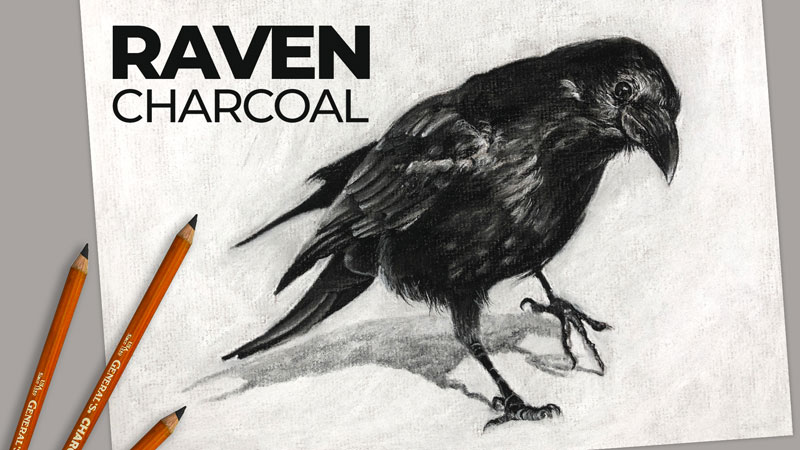This image showcases a detailed charcoal drawing of a raven, centered against a predominantly white background with some gray shading. The raven, rendered with thin white accents around its eyes and ears, sports sleek, textured feathers and is depicted in a perched stance with its right foot firmly on the ground and its left foot slightly raised, just touching the surface. Defined shadows under its feet accentuate its presence. On the top left of the image, the bold, capitalized text "RAVEN" appears above a finer-font "CHARCOAL," both serving as titles for the drawing. To the left of the artwork rests a trio of yellow pencils with black tips, likely the tools used to create the intricate details of the bird. Intricate, long toes and white specks interspersed on the raven’s body add to the lifelike portrayal of the bird.